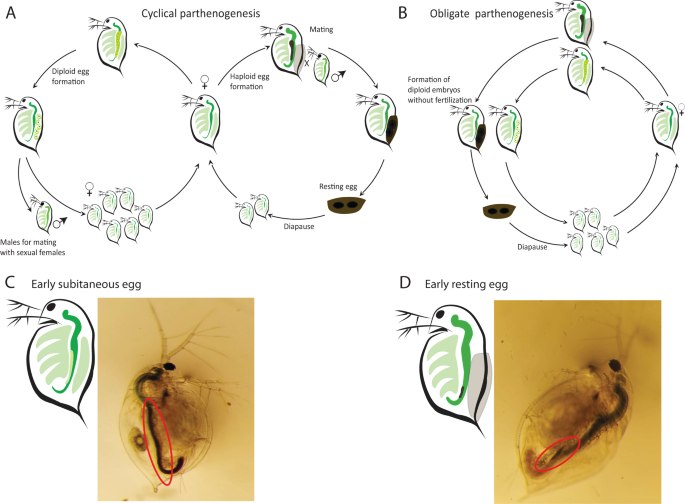This image, set against a plain white background, is a detailed biological diagram focused on different stages of a flea-like organism's life cycle, labeled from A to D. The diagram is divided into four sections without actual borders separating them:

1. **Section A: Cyclical Parthenogenesis** - This section features two interconnected circular flowcharts with arrows indicating a repeating cycle. It outlines various stages including mating, resting eggs, haploid egg formation, and diploid egg formation. Symbols for male and female genders are included, highlighting the cyclic nature of reproduction.

2. **Section B: Obligate Parthenogenesis** - Located in the upper right, this section contains a single circular flowchart with an inner circle also marked by arrows. It describes the formation of diploid embryos without fertilization and mentions diapause, indicating a part of the organism's life cycle that proceeds without mating.

3. **Section C: Early Subcutaneous Egg** - Situated in the lower-left corner, this section combines a diagram with a real-life photo of the organism, displaying a semi-transparent flea-like insect with visible internal structures. A red circle highlights a specific part of the image, pointing out a critical feature in subcutaneous egg development.

4. **Section D: Early Resting Egg** - In the lower right, this section also merges a diagram with a photograph, similar to Section C. It shows another view of the flea-like insect with a red circle emphasizing a section, which likely represents an egg at the early resting stage.

Each section is meticulously detailed, providing a comprehensive visual and textual breakdown of the organism's reproductive and developmental stages.